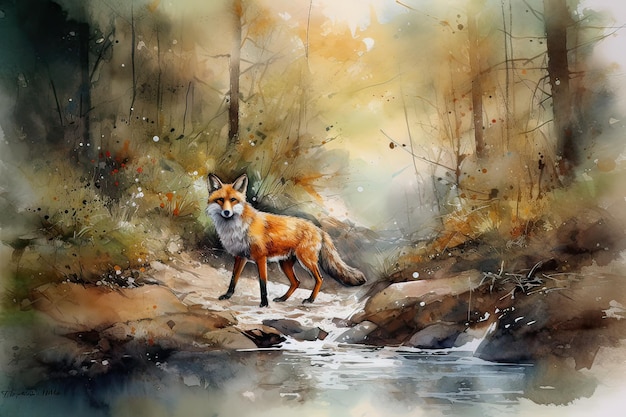This detailed watercolor or mixed-media painting captures a red fox standing in front of a stream, exuding a sense of cautious curiosity. The fox, adorned with a striking orange coat, a white underbelly, and black feet, is depicted forward-facing with pointy ears perked up, and white detailing on its neck, whiskers, and cheeks. The scene, set in a fall woodland, features a barren forest in the background, with muted greens, yellows, and browns blending seamlessly. Large boulders and rocks are scattered across the creek bed, with sparse flowers and bushes adding subtle bursts of color. The overall composition of muted tones and blended shades enhances the serene yet alert demeanor of the fox, standing slightly left of the center, appearing ready to leap into action at any moment.